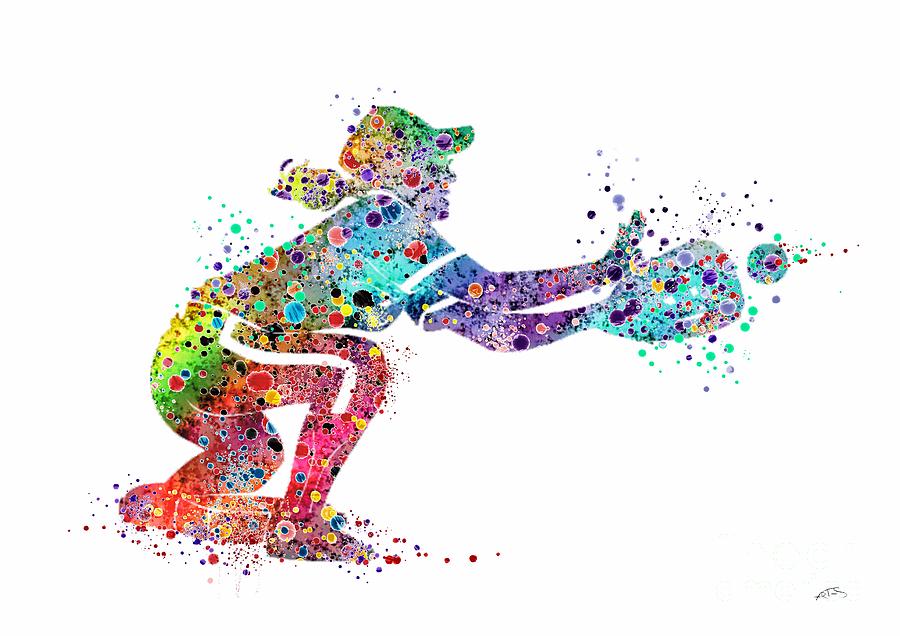This vibrant painting features an artistic depiction of a female baseball player poised to catch a ball. The image, set against a very light, off-white, rectangular background approximately four inches high by six inches wide, showcases the player squatting atop a catcher's mound, facing the right. Her body is dynamically posed with knees bent and an arm extended forward, ready to receive the ball approaching from the right. Decorative details include a ball cap transitioning from green to yellow with a yellow ponytail emerging from the back. The playful use of colors defines her form: her glove and the ball are blue, her arms and face are purple, her shirt transitions from blue to brown, her pants shift from green at the back to pink towards the legs, with an added white stripe on the right side. The entire figure is lavishly adorned with colorful splatters and circles that contrast with and complement the base colors of the silhouette, creating an eye-catching, ornamented design.